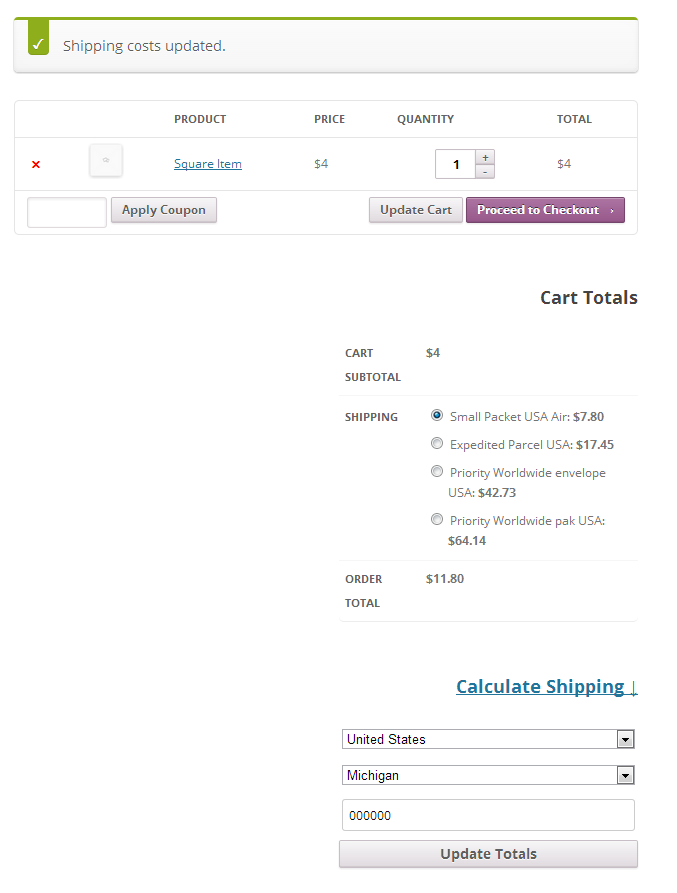The screenshot shows an order page detailing shipping costs. At the top, there is a light gray banner that reads "Shipping costs updated," accompanied by a check mark. Below this banner, there are four headings: Product, Price, Quantity, and Total.

- Under Product, "Square Items" is listed.
- Under Price, "$4" is noted.
- Under Quantity, the number "1" is selected.
- The Total column reflects a price of "$4."

Beneath these headings, there is a blank text box labeled "Apply coupon" with an "Update cart" button to its right. Next to this is a prominent purple button labeled "Proceed to checkout."

On the right-hand side of the page, there is a column titled "Cart totals." This section shows:
- Cart Subtotal: $4
- Shipping options with radio buttons:
  - The selected option is "Small Packet USA Air" costing $7.80.
  - Other options include:
    - "Expedited Parcel USA" for $17.45
    - "Priority Worldwide Envelope USA" for $42.73
    - "Priority Worldwide Pack USA" for $64.14

The Order Total is displayed as $11.80.

Below this, there is an option to "Calculate shipping" in blue, underlined text, followed by a dropdown box with "United States" selected. Another dropdown shows "Michigan," and next to it is a text box with the value "000000." At the bottom of the column, there is an option labeled "Update totals."